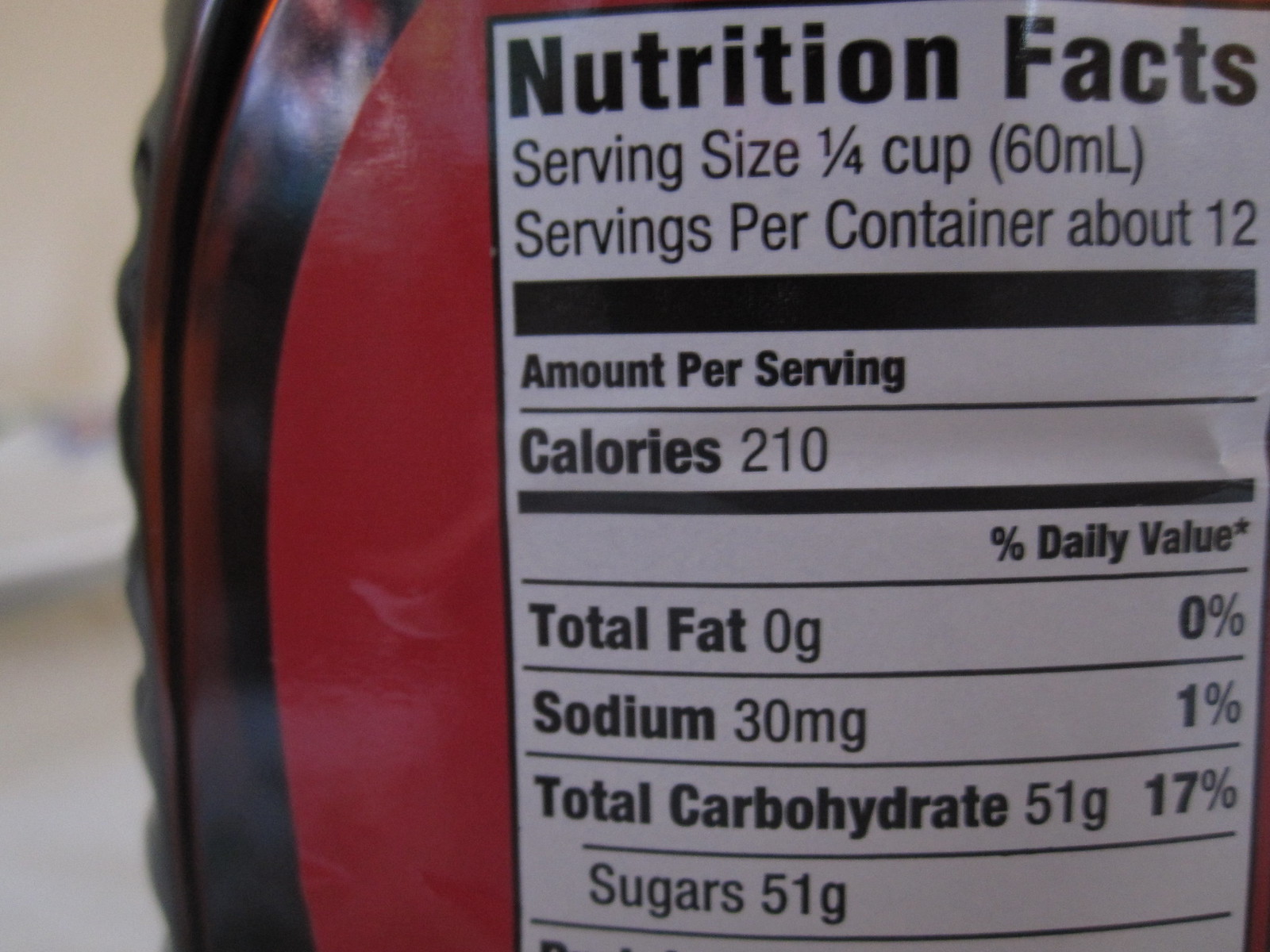This close-up image focuses on a section of a nutrition label on the back of a syrup bottle. The left side of the nutrition label features a hint of red, part of the overall design. Beyond the red area, a dark black and brown color can be seen, which might represent either the bottle or the syrup inside. The nutrition label clearly displays the text "Nutrition Facts" in black. Beneath this heading, the serving size is stated as one-fourth cup (60 milliliters), with approximately 12 servings per container. The breakdown per serving includes: 210 calories, 0 grams of total fat (0% daily value), 30 milligrams of sodium (1% daily value), 51 grams of total carbohydrates (17% daily value), and 51 grams of sugars.